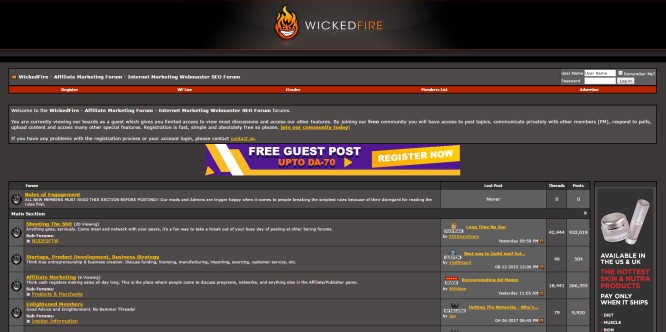The image depicts a promotional page for a product or service named "Wicked Fire." The title "Wicked Fire" is stylized with the words "Wicked" and "Fire" in two distinct colors to create a striking visual contrast. At the top of the page, there is a logo featuring a devilish figure with its head engulfed in flames. The devil appears to be wearing a mask, giving it an uncanny and mysterious appearance.

The rest of the page is cluttered with text and graphics that are too small to read clearly. Positioned centrally is an advertisement offering "free guest posts" with the promise of "up to DA-70." It's unclear if the phrase "up to" is an error or intentional. Below this offer, a prominent "Register Now" call to action is highlighted with arrows directing attention to it. There is a list of six items below the registration prompt, written in yellow text with accompanying white descriptions, though these details are too small to decipher.

On the right side of the page, there is an image featuring an assortment of products indicated to be available in the US and UK. The products include what appear to be a canister and a tube, although the exact nature of these items remains unidentified. The overall design of the page is visually busy, with many elements competing for attention.